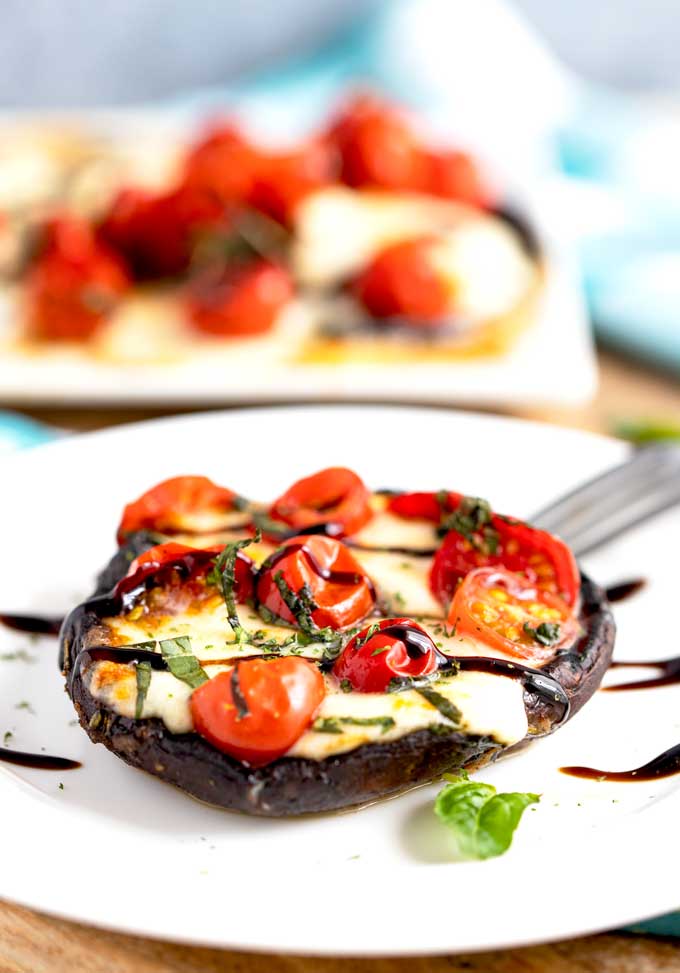The image depicts a meticulously crafted culinary creation, possibly prepared for a fine dining experience, served on a simple white plate. At the center of the plate is a small, elegantly presented dish featuring an upside-down, baked mushroom cap with dark, singed edges, resembling an artistic miniature pizza. The mushroom is topped with a layer of melted white cheese, creating a rich and creamy appearance. Surrounding the cheese are delicately placed slices of juicy cherry tomatoes, numbering seven. Scattered among the tomatoes are small, fresh green leaves, likely basil, adding a vibrant touch of color. The dish is finished with a drizzle of a brown sauce, possibly vinaigrette, artfully zigzagged across the top. A fork rests near the upper right side of the plate, hinting at a ready-to-eat meal. In the background, there's another dish, blurred out with a strong bokeh effect, further emphasizing the close-up focus on the main gastronomic artwork.